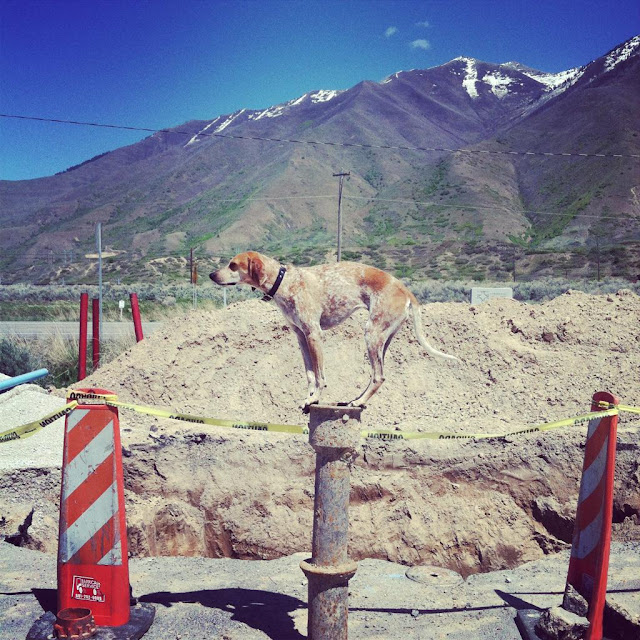This is a color photograph capturing an industrial or construction site set against a stunning natural backdrop. Central to the image, a thin, wiry brown and white dog stands confidently on top of a metal post emerging from the pavement, facing left and adorned with a black collar. Below, a pit is encircled by bright orange pylons with white and orange stripes, interconnected by yellow caution tape that bears black caution warnings. The background reveals a vast expanse of dirt or sand, indicating extensive digging, possibly for highway construction. Red poles sprout from the ground on the left side, adding to the maze of construction elements. The scenery transitions smoothly from the bustling site to a serene, partially snow-capped mountain range under a clear, gradient blue sky accented by a few wispy clouds. Scattered green trees dot the sides of the mountain, complemented by a series of telephone poles and wires stretching across the horizon. The overall palette includes dark orange, white, yellow, green, purple, blue, brown, beige, red, orange, burgundy, and gray, painting a vivid and detailed scene that balances human activity with the tranquility of nature.